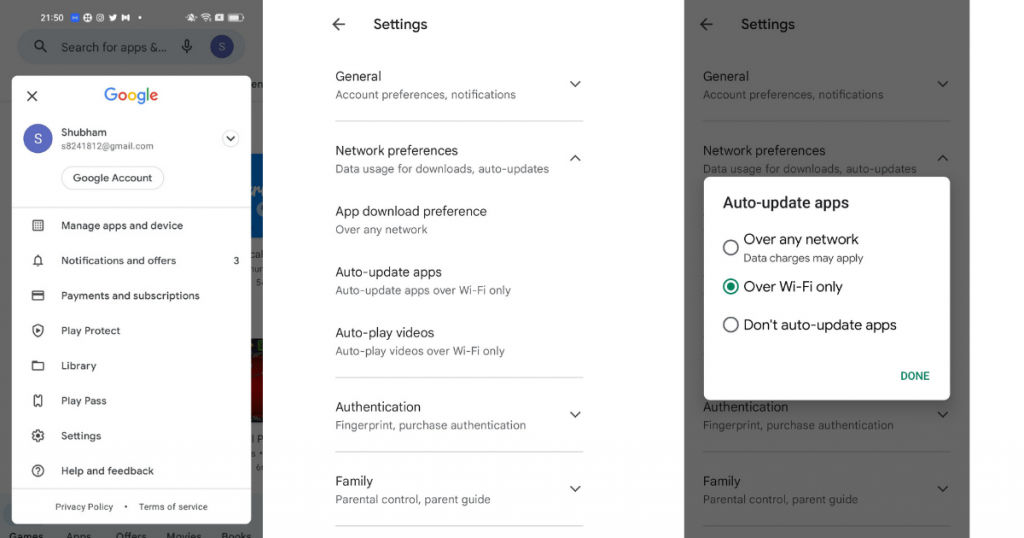Here is the cleaned-up and detailed caption for the image:

---

The image showcases three consecutive screenshots of a smartphone interface. 

1. **First Tab: Google Play Store Account Overview**  
    - At the top, the screen displays the current time (2:50) and several notification icons.
    - Beneath the search bar, which features a white "Google" search button, the user's account details are highlighted: "Shubham" with the email address "shubham241812@gmail.com" and a dropdown arrow.
    - Below this, there's a series of menu options: "Manage apps and device," "Notifications," "Offers," "Payments and subscriptions," "Play Protect," "Library," "Play Pass," "Settings," and "Help and feedback." 

2. **Second Tab: Google Play Store Settings**  
    - This tab displays several sections under the settings menu.
        - **General**: Account preferences and notifications with dropdown arrows for more options.
        - **Network Preferences**: 
            - Data usage for downloads.
            - Auto-update apps, with a dropdown arrow to select preferences.
            - App download preference for any network or Wi-Fi only.
            - Auto-play videos set to Wi-Fi only, showing as "Off" for the current status.
        - **Authentication**:
            - Fingerprint purchase authentication.
        - **Family**:
            - Parental controls and parent guide.

3. **Third Tab: Auto-update Apps Setting**  
    - The tab displays a prompt focusing on the "Auto-update apps" settings within a large white box.
    - Users can choose from three options:
        - "Over any network (data charges may apply)"
        - "Over Wi-Fi only" (currently selected, marked with a green checkmark)
        - "Don't auto-update apps."
    - A "Done" button is visible at the bottom in green color, indicating that changes can be confirmed.

---